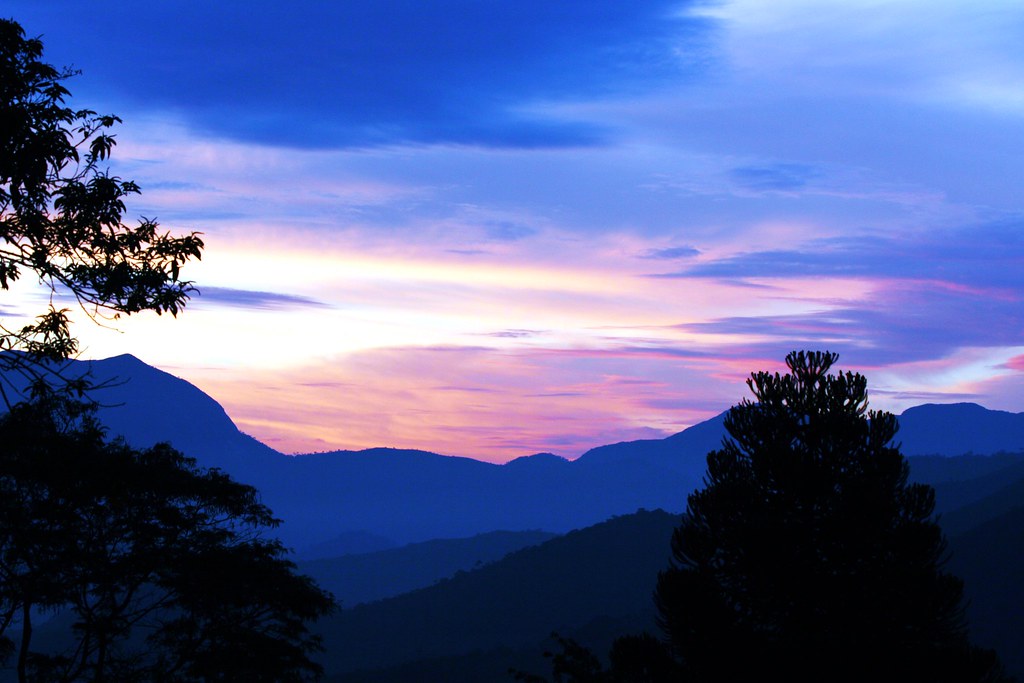This image captures a mesmerizing sunset landscape dominated by a vivid sky and deeply shadowed foreground. The sky takes center stage, painted in a breathtaking gradient from dark blue at the top to light blue, then transitioning into shades of purple, pink, orange, yellow, and a touch of gold near the horizon. The clouds reflect this dynamic palette, displaying hues of dark blue, light blue, white, and pink where they catch the sun’s last light. Below this stunning skyscape, the mountains and evergreen trees stand as dark silhouettes, almost black against the radiant backdrop. The largest evergreen tree is prominently in the foreground, with additional trees to the left, allowing glimpses of the colorful sky through their branches. The overall setting suggests a serene yet dramatic evening scene where the vibrant sky sharply contrasts with the darkened, indistinct shapes of the landscape below.